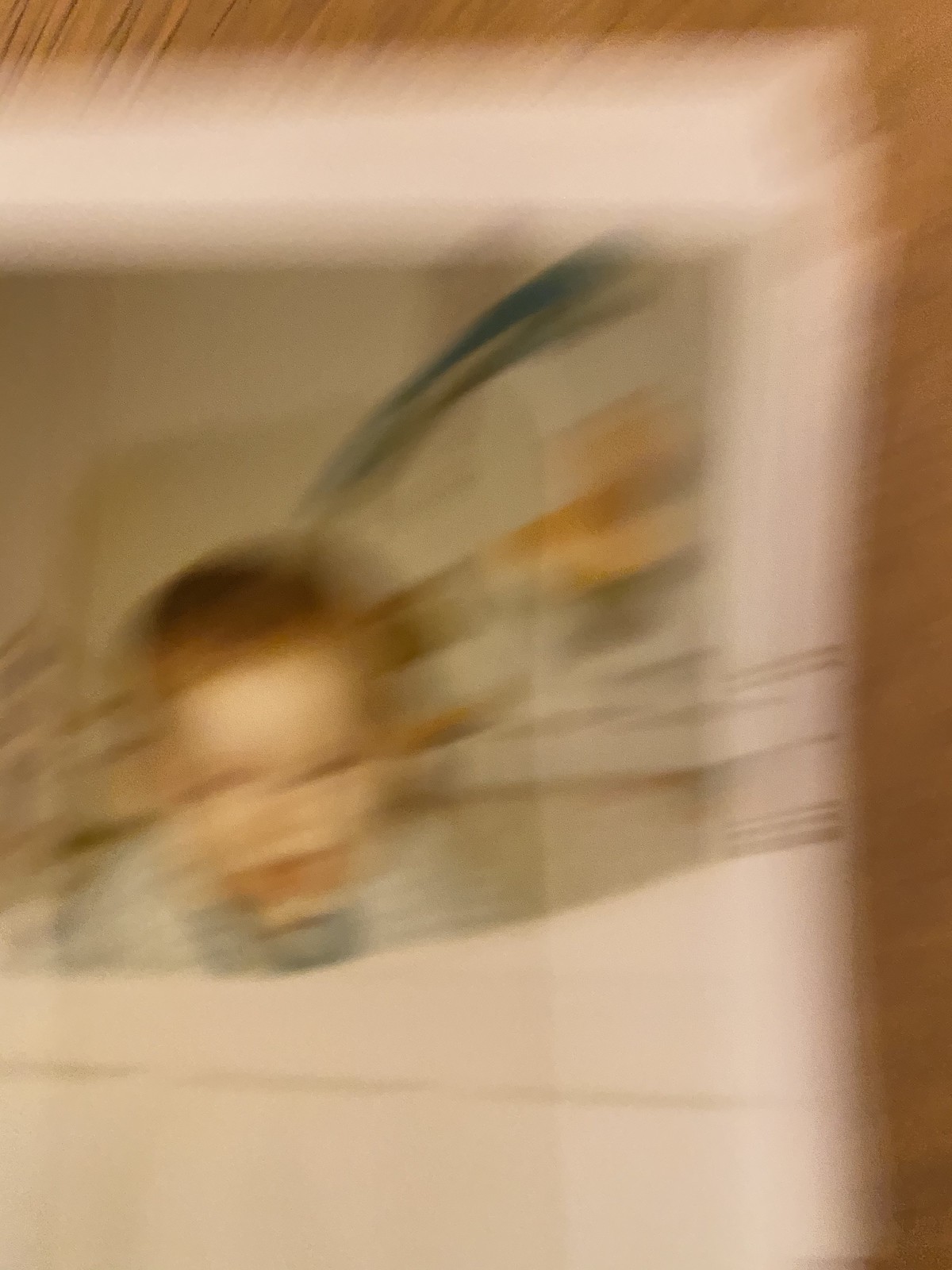This image captures an extremely blurred photograph taken of another photograph laying on a wooden table. The primary colors in the image are brown, white, and various shades of blue. The photograph within the photograph appears to be a young white toddler with short, possibly red or light brown hair, wearing a light blue shirt. The child is looking straight at the camera with an open mouth and a smile. There's a significant amount of motion blur, indicating the camera moved while capturing the image, resulting in visible streaks and lines, particularly a darker blue streak coming from the top of the child's head to the top right. The old photograph has a white border on the top and right side, with a wider white border along the bottom, hinting it might be a Polaroid. Behind the photograph, you can faintly see the wooden table, characterized by diagonal grains in various shades of brown.